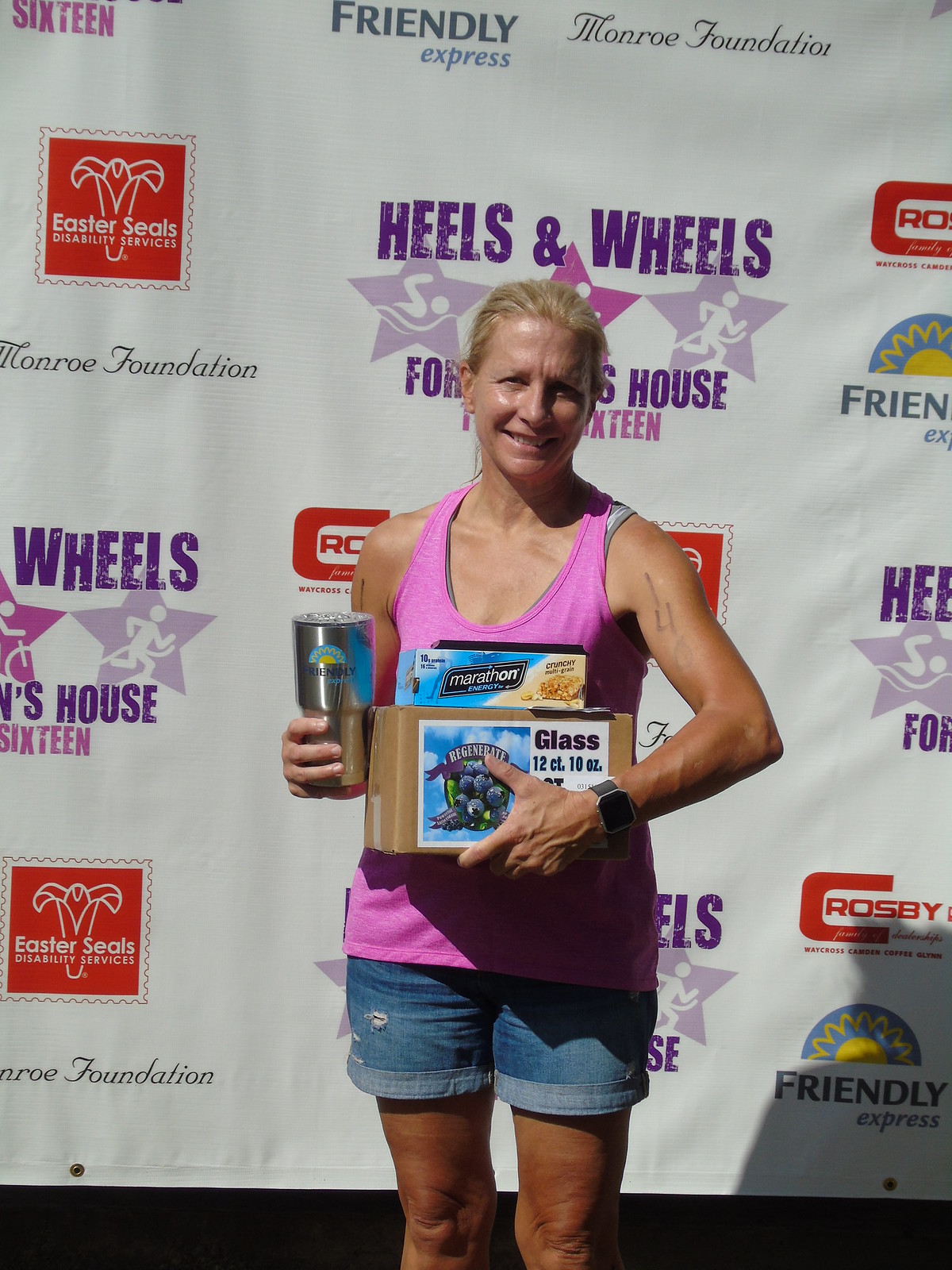This rectangular outdoor photograph, taken during the daytime, features a mid-aged, slightly older Caucasian woman, approximately in her 50s, standing in front of a large white banner adorned with various sponsor logos, including Monroe Foundation, Friendly Express, Easter Seals, and Heels and Wheels. The banner includes a prominent red square with white text and different purple text elements.

The woman, captured from about the knees up, has her blonde hair pulled back into a ponytail or neatly secured behind her head. She is smiling and squinting, likely due to the bright sunlight. She is dressed in a pink tank top layered over a gray sports bra and wearing cut-off jean shorts that are rolled at the hem and slightly distressed.

In her left arm, bent at the elbow, she holds a cardboard box with a white label adorned with blue and purple designs, including an image of blueberries and the text "glass 12 count 10 ounces." Atop this box, she balances a smaller box labeled "Marathon Energy," presumably containing protein bars. Her right hand grasps a large stainless steel tumbler branded with "Friendly Express."